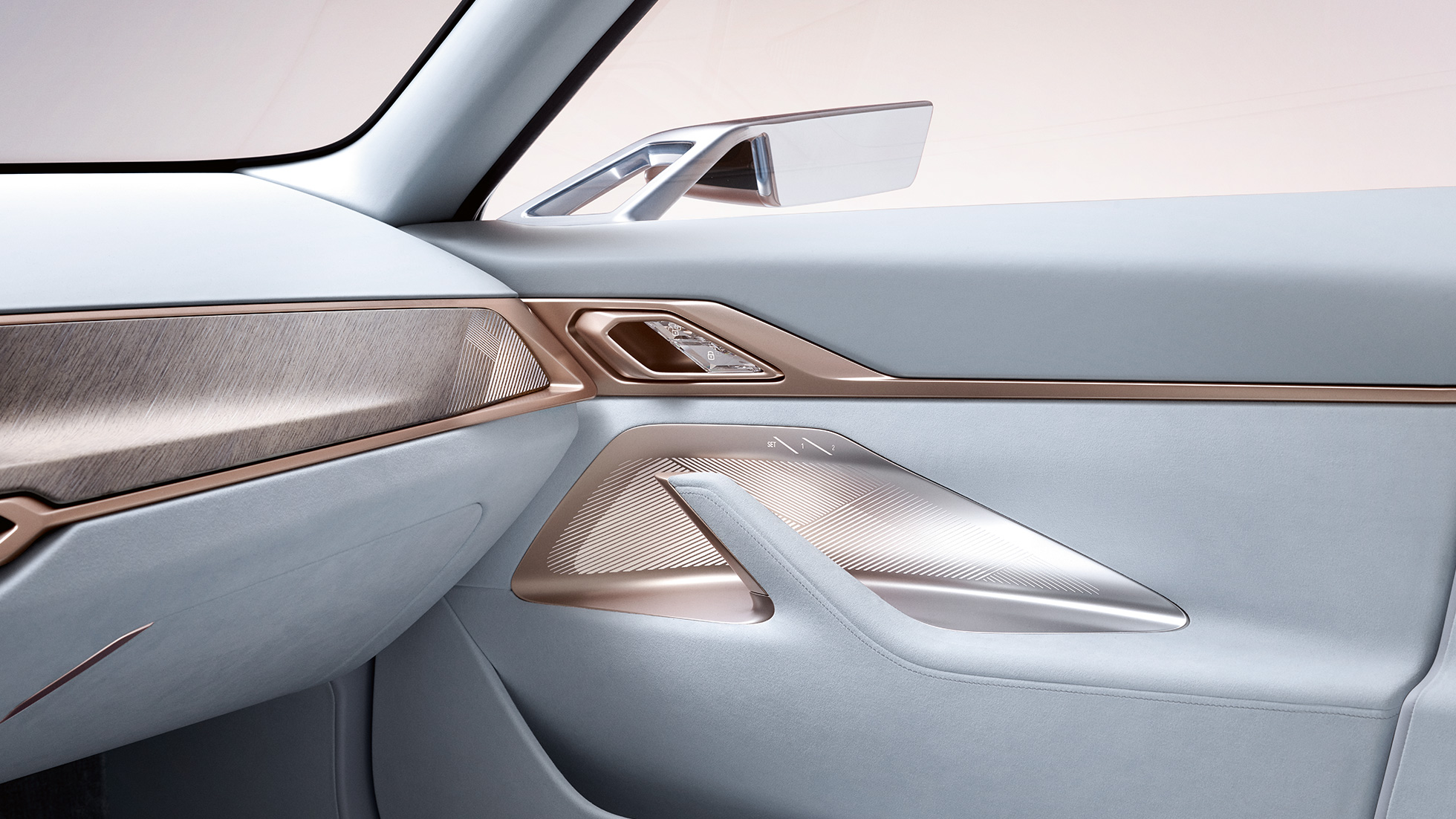This color photograph captures the luxurious interior of a modern vehicle, emphasizing a sleek design and high-end finishes. The passenger side dashboard is a light silverish-blue color, complemented by shiny rose gold accents that run down the middle and across various touchpoints, including the rectangular panel and handle on the passenger side door. The door panel itself includes functional elements such as buttons for locking and unlocking the door, as well as window controls. The driver's side door handle also features a light silverish-blue color, harmonizing with the overall aesthetic. Outside the passenger window, a silver chrome side mirror reflects the contemporary design of the car. The entire vehicle interior appears very clean, new, and modern, with an emphasis on luxury, possibly captured in a showroom setting given the nondescript view beyond the windows.